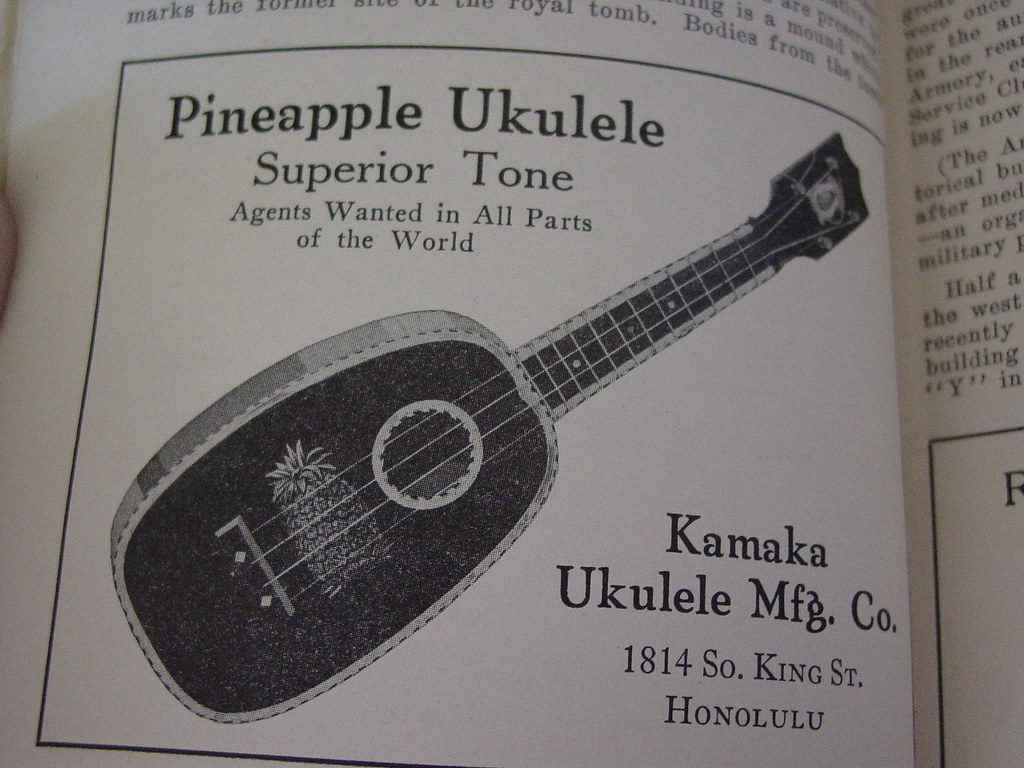The image features a black and white photograph of a newspaper or pamphlet advertisement for a ukulele. The focal point of the ad is a detailed illustration of a "Pineapple Ukulele," emphasizing its "Superior Tone." The text prominently states "Agents Wanted in All Parts of the World," and provides details about the manufacturer, "Kamaka Ukulele Manufacturing Co." located at "1814 S. O. King Street, Honolulu." The ad occupies the lower half of the page, with neighboring text and print suggesting it's part of a larger publication. A finger is visibly holding the page open in the top left corner, indicating that this image is a photograph of someone holding the pamphlet or newspaper.